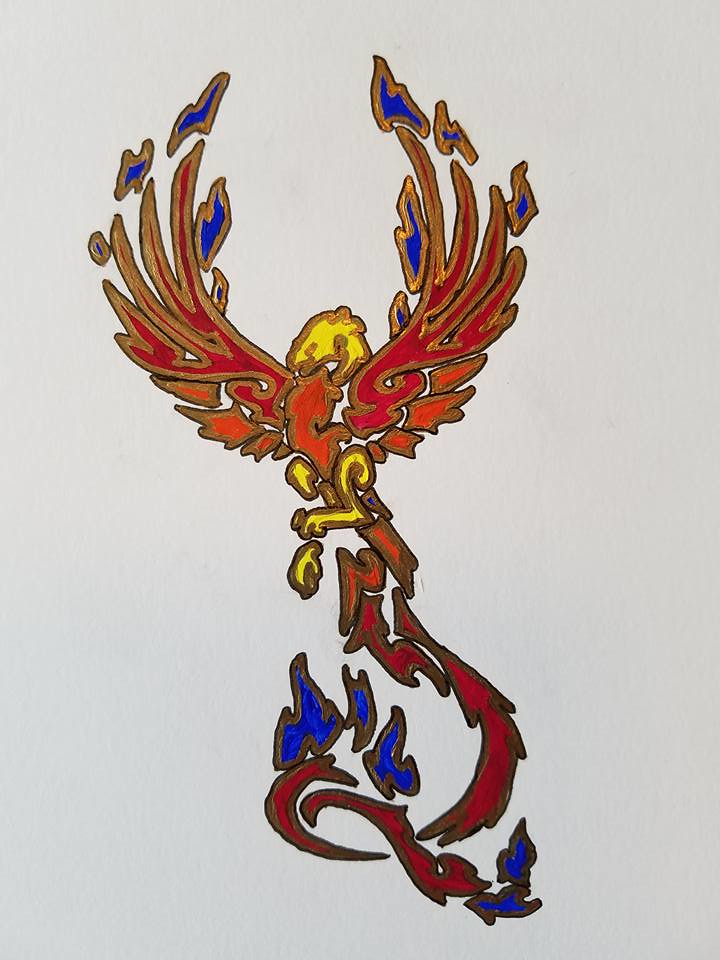This abstract drawing, seemingly rendered with ink, magic marker, or colored pens, showcases a dynamic blend of shapes and colors. Dominating the top portion of the piece are what appear to be outstretched wings of a bird, though the abstraction leaves some room for interpretation. These wings, resembling an upward-curving letter U, are vividly colored in red with light brown outlines. At the very top, blue feathers, also outlined in brown, provide a striking contrast. The lower section continues the theme, featuring more dark red shapes bordered with brown, alongside royal blue forms, similarly outlined in brown. These elements together create a flowing, squiggly design that evokes the image of a partially rendered letter D, contributing to the overall sense of fluidity and motion in the artwork.